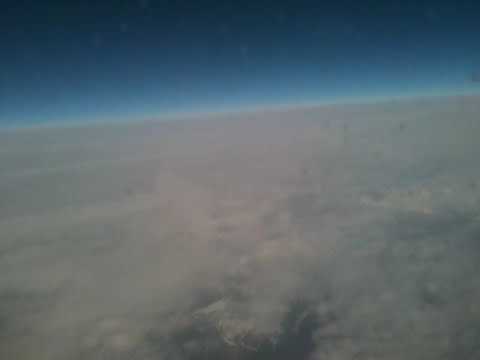The image appears to depict a serene scene likely taken from an airplane window. The lower portion of the image is dominated by a tan-colored sandy area that resembles a beach, extending towards the horizon. Above it, a beautiful, cloudless blue sky stretches across the frame. In the middle section, the horizon is marked by a fuzzy, cottony layer of white clouds, visible from an aerial perspective. There is a distinct gradient in the sky's color, transitioning from lighter to darker blue as you look upward. Small splotches scattered throughout the image suggest it was captured through a window, possibly slightly dirty. The overall impression is one of tranquility, with the sandy expanse below, a clear sky above, and a harmonious meeting of the two in the middle, with only the faintest hint of cloud cover.